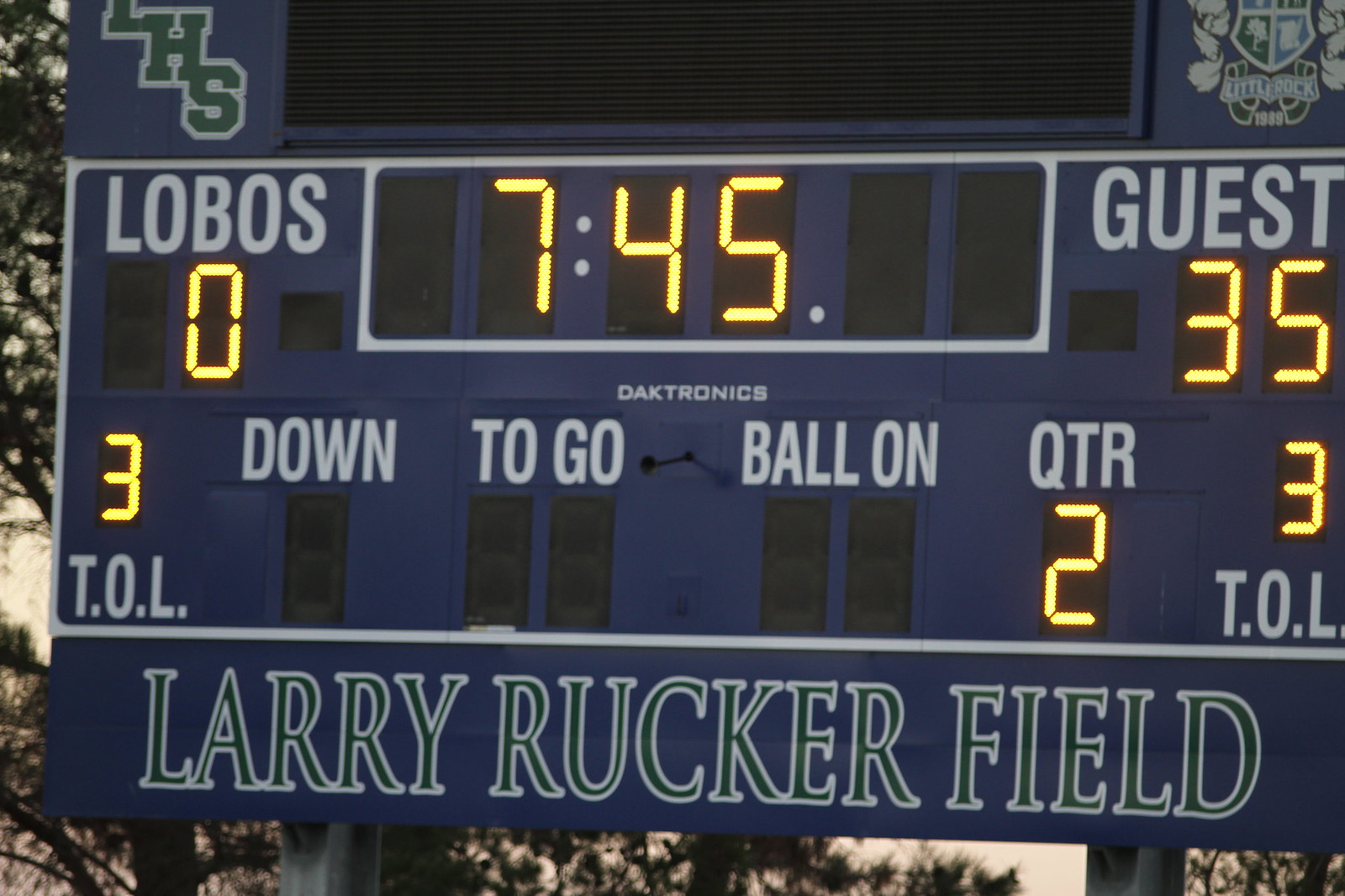The image focuses on a blue scoreboard with digital readouts in a stadium, displaying detailed information likely for a football game. At the top of the scoreboard, slightly cut-off logos include the initials "LHS" in light blue font and a crest representing Little Rock. Below these, the name "Larry Rucker Field" appears in green, all-capital text with a white outline. The scoreboard displays "Lobos" to the left and "Guest" to the right. The current score is 35 for the Guest team and 0 for the Lobos. The game is in the second quarter, with 7:45 left on the clock. Both teams have three timeouts left. Additional readouts on the scoreboard indicate details such as "TOL" (timeouts left), "down", "to go", "ball on", and "quarter". Behind the scoreboard, trees are visible, indicating a twilight setting.